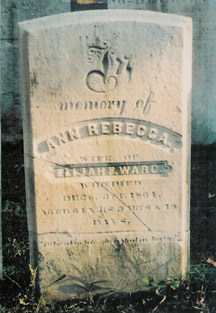This is an outdoor daytime photograph of an old-fashioned grey stone headstone, which is slightly grainy and not very high quality. The headstone, likely made of concrete, displays an inscription at the top that reads "In memory of" in cursive letters. Beneath this, "ANNE REBECCA" is inscribed in capital letters, followed by the designation "wife of Elijah B. Ward," although one source mentions Elijah H. Ward. The exact date of death is somewhat obscured, but appears to say "December 1801." The headstone bears a midline crack extending from the left side down towards the right corner. This weathered memorial stands on a bed of green grass, surrounded by some dirt, leaves, and weeds. Behind the headstone, there is a grey wall or concrete structure, enhancing the solemn atmosphere of the scene.